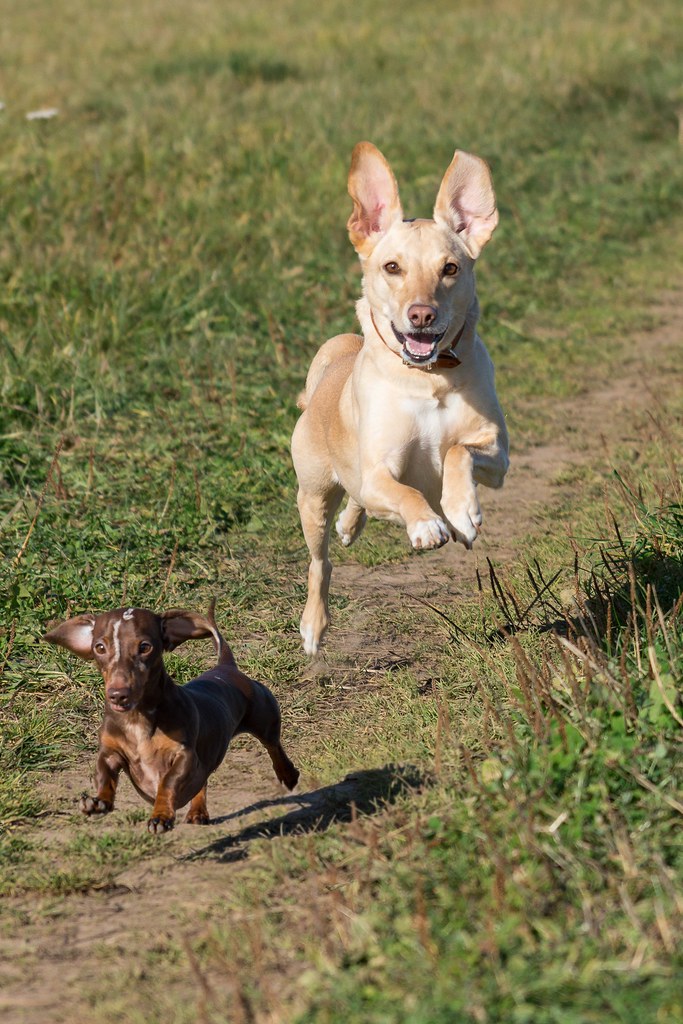Two dogs are seen playing chase in a vibrant photograph. The dog in the lead is a chocolate brown with hints of orange around its legs, boasting a long body and short legs. Behind it, a lighter-colored dog, with three legs off the ground, appears to be in mid-stride. This dog has blonde and tan fur, a light brown nose, and expressive brown eyes. Its ears stand straight up, revealing pink inner linings. With an open mouth showcasing its white teeth and pink tongue, the dog exudes a joyful expression.

The ground beneath them is a mixture of green grass, with patches turning yellow towards the background, interspersed with darker green and brown areas in the foreground. A dirt path winds through the middle of the grassy field. The shadow of the leading dog stretches across the grass, adding depth to the scene. Among the grass, thin, weed-like brown plants are visible, bathed in sunlight that enhances the crisp, clear quality of the image.